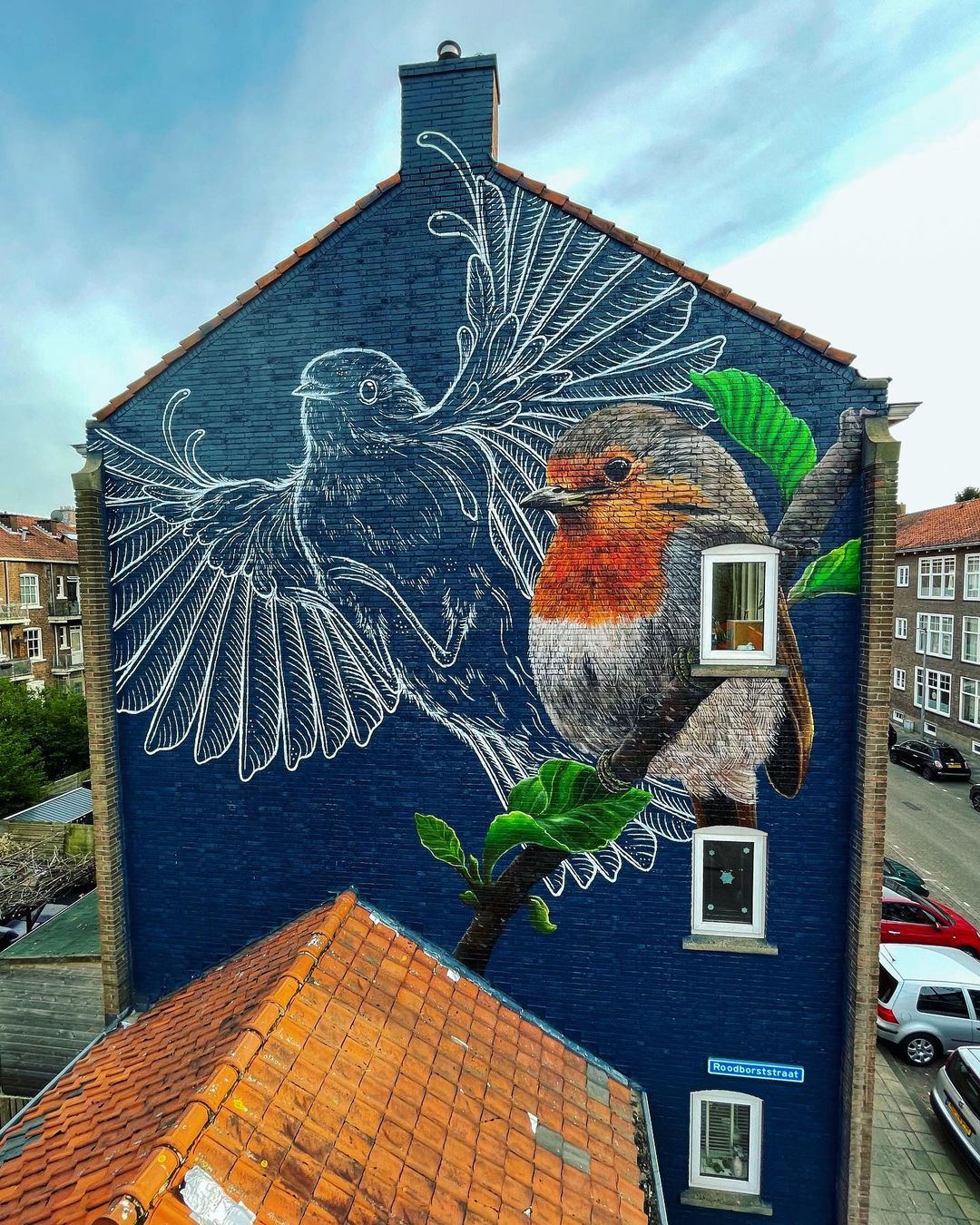This photograph captures a striking mural on the side of a tall, approximately four-story apartment building in a neighborhood. The building, which is the main focus of the image, is painted a deep navy blue and features two bird illustrations. One bird, perched on a painted dark brown branch with green leaves, is depicted in full color with an orange face, darker feathering on the head, and white fur near the legs and belly. The other bird, a large white outline, appears to be flying just behind the first bird and takes up nearly the entire wall. Down the right side of the building, there are three small white window sills. Above the scene, the sky is a clear blue, and in front of the mural, there's a building with an old orange-tiled roof, adding a contrasting element. To the right, a row of parked cars lines the sidewalk. The mural, vivid in its detailing, breathes life into the surrounding urban environment.